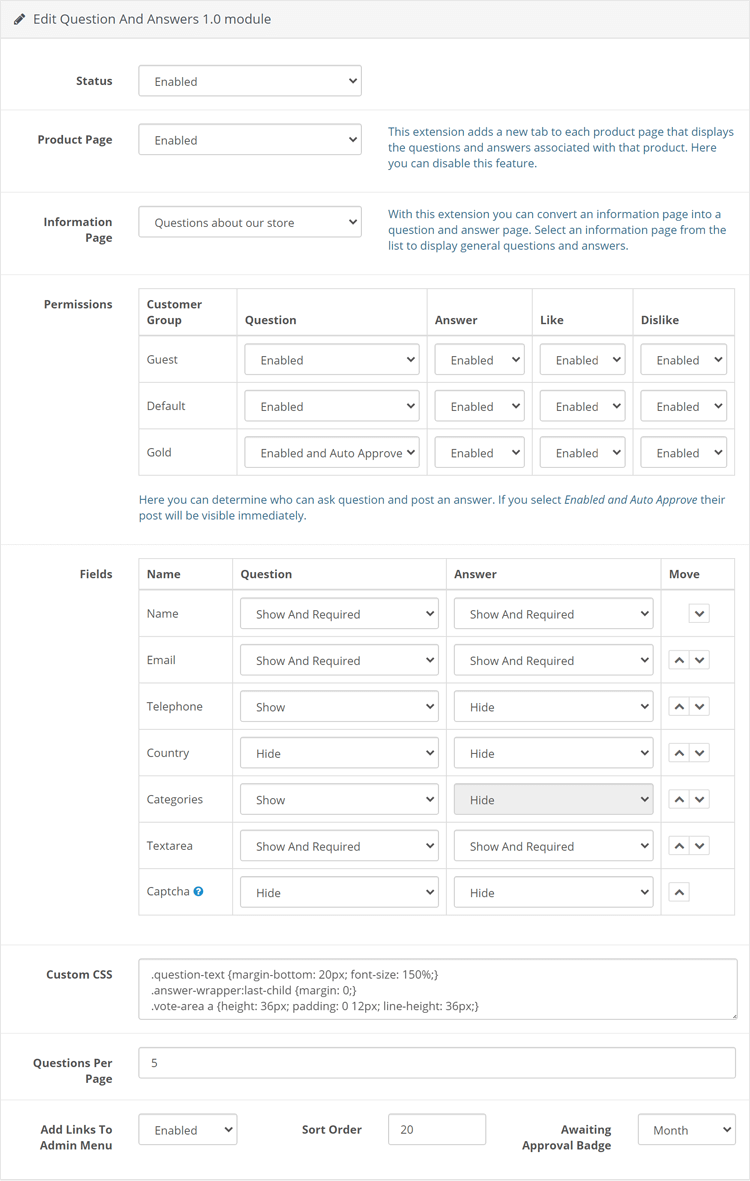The image depicts an all-white background user interface for an "Edit Question and Answers 1.0" module. 

In the top-left corner, there is a pencil icon accompanied by the text "Edit Question and Answers 1.0 module". 

Below this, the interface is divided into various sections:

1. **Headers Section**:
   - **Status**: A drop-down box with "Enabled" selected.
   - **Product Page**: Another drop-down box also set to "Enabled". To the right, in blue text, it reads: "This extension adds a new tab to each product page that displays the questions and answers associated with that product. Here you can disable that feature."
   - **Information Page**: On the left, a header labeled "Information Page"; to the right, a drop-down box labeled "Questions About Our Store" with accompanying blue text to the right.

2. **Permissions Section**:
   - A header labeled "Permissions" with a table on the right. The table headers read: "Customer Group", "Question", "Answer", "Like", "Dislike". The first column lists: "Guest", "Default", "Gold" with drop-down boxes in each square set to "Enabled".
   - Below, another sentence in blue text.

3. **Fields Section**:
   - A header labeled "Fields" followed by a table with headers "Name", "Question", "Answer", "Move". The first column details: "Name", "Email", "Telephone", "Country", "Categories", "Text Area", "Captcha" with corresponding drop-down boxes in each cell.
   - Below this table, "Custom CSS" is noted with a text entry selection box.

4. **Settings Section**:
   - A header labeled "Questions Per Page" with a text entry box containing the number "5".
   - "Add Links to Admin Menu" is displayed with a drop-down box set to "Enabled".
   - A "Sort Order" label with a text entry box showing the number "20".
   - To the right, "Awaiting Approval Badge" with a drop-down box labeled "Selected Month".

Each section is clearly defined and structured, with detailed settings for customization and management of the "Edit Question and Answers" module.